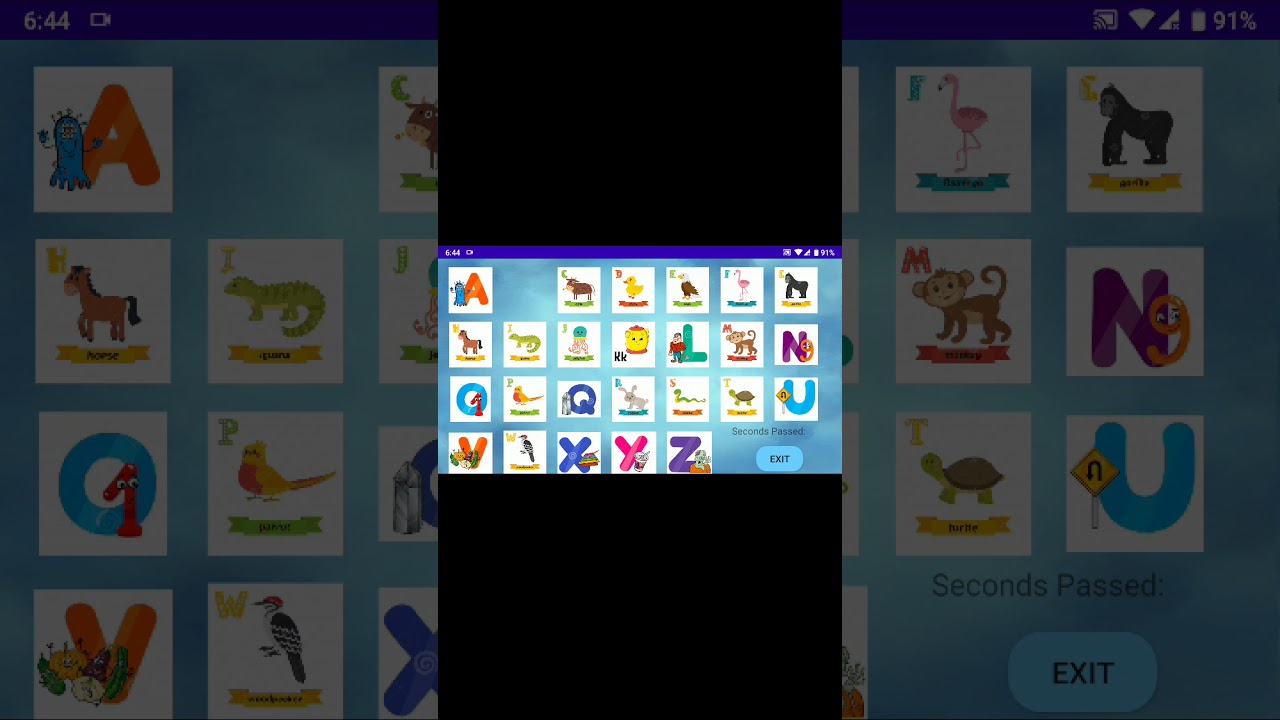The image is a screenshot of a digital device, likely a tablet or a mobile phone. The central focus of the screenshot is an inset image, which appears as a smaller version of the main background image, bordered by two black rectangles on the top and bottom. At the top of the image, there's a dark bar with white text, indicating the time as 6:44. This bar also includes a camera icon on the left and a series of icons on the right, such as a streamcasting icon, a Wi-Fi symbol, reception bars, and a battery indicator showing 91% charge.

The main and inset images display a collection of alphabet cards, with each card featuring a letter alongside an illustration of an animal, creature, or item that represents that letter. For example, 'A' is accompanied by an amoeba, 'M' by a monkey, 'N' by the number 9, 'T' by a turtle, and 'P' by a parrot. The entire setup suggests an educational or learning application, with the inset image possibly being a zoomed-in view for clarity or emphasis.